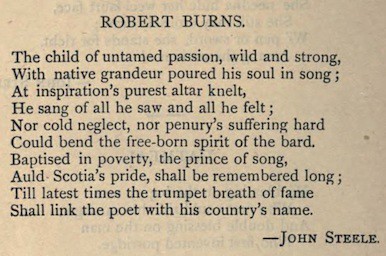The image depicts an aged, slightly browned page from a book or newspaper, with the words from the opposite side faintly bleeding through. At the top of the page, the title "Robert Burns" is prominently displayed. The text, attributed to John Steele at the bottom right, is a poetic tribute to Robert Burns. The passage reads: 

"The child of untamed passion, wild and strong, with native grandeur, poured his soul and song. At inspiration's purest altar knelt. He sang of all he saw and all he felt. Nor cold neglect, nor penuries suffering hard, could bend the free-born spirit of the bard. Baptized in poverty, the prince of song, Old Scotia's pride shall be remembered long. Till latest times the trumpet breath of fame shall link the poet with his country's name." 

This eloquent excerpt highlights Burns' spirited nature and enduring legacy, celebrating his contributions to poetry and his deep connection with Scotland.